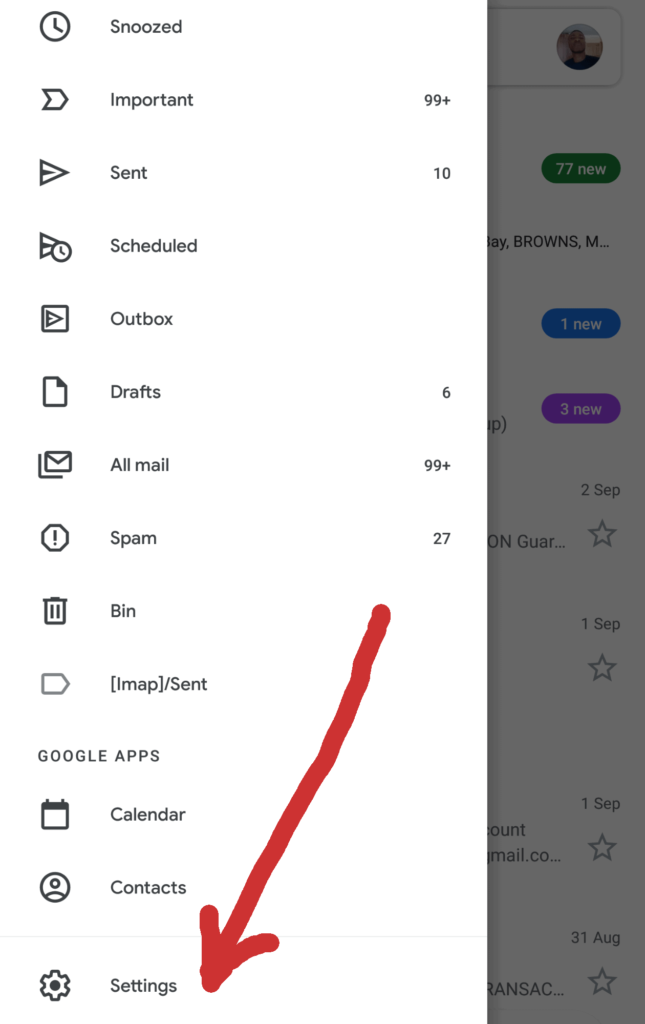In this image, we see the options menu of an email application has been activated, revealing an extensive list of categories and features on the left side of the screen. The menu items are displayed in a vertical list with options such as "Snoozed," "Important," with a significant number of messages marked as important tallying over 99, "Sent" containing 10 messages, "Scheduled," "Outbox," "Draft" with 6 drafts, "All emails" also exceeding 99 messages, "Spam" with 27 messages, and "Bin." Below these, options like "Calendar" and "Contacts" are visible, and at the very bottom, there is a setting labeled "Settings."

To the right, the main panel of the application shows a darker background and is arranged in the foreground. Here, we can see the profile icon of the user and a list of emails organized by date, starting with the most recent. The first email is marked with "77 new" in green, the second with "1 new" in blue, and the third with "3 new" in purple. Other emails are dated 2nd September, 1st September, and 31st August, continuing in reverse chronological order. The dates extend back to February 8th.

An error indicator is notably present, drawn from the right side in red, pointing towards the "Settings" option, presumably marking an issue that needs attention. All text within this interface is displayed in black font, ensuring clarity and readability.